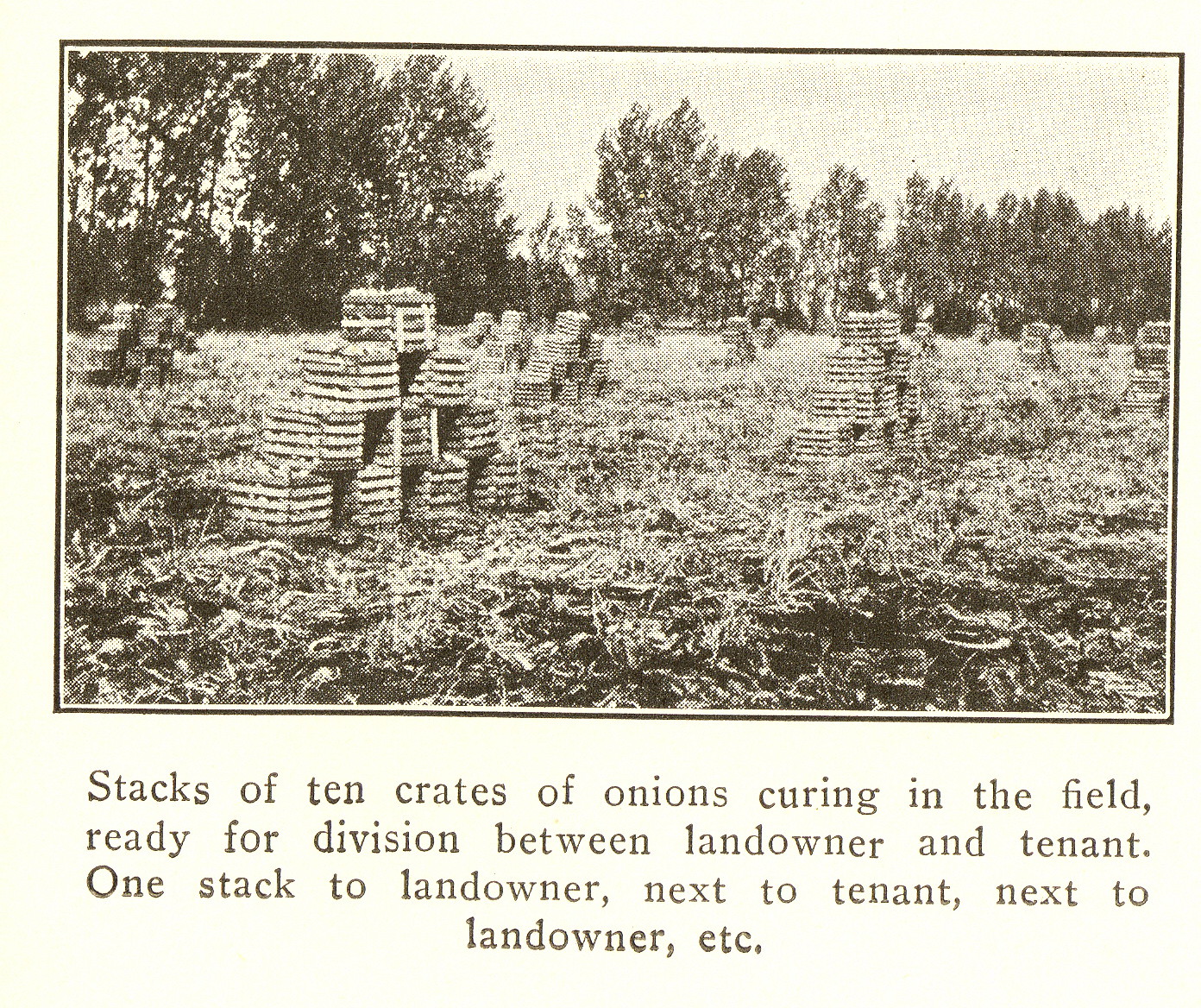The vintage black-and-white photograph, occupying more than three-quarters of the top portion of an image with a black border, exudes a nostalgic charm reminiscent of old newspaper prints, complete with crosshatch marks from the newsprint. The scene depicts a spacious field with grass covering the ground and a line of trees in the background. Dominating the field are stacks of crates arranged in a stair-like pattern, each composed of 10 crates, believed to contain onions. These crates are meticulously piled in clear groups indicating forthcoming division. Beneath this evocative image, a caption in black text on a cream background states: "Stacks of 10 crates of onions curing in the field, ready for division between landowner and tenant. One stack to landowner, next to tenant, next to landowner, etc." This text clarifies the purpose of the crates and the systematic, alternate allocation between landowner and tenant, providing a historical peek into agricultural practices.